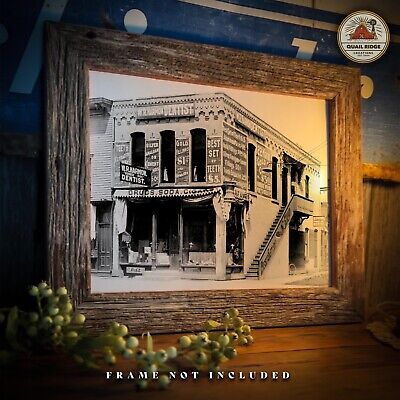This detailed advertisement photo features a framed, black-and-white artwork depicting a turn-of-the-century two-story country store. The framed piece, likely a pencil drawing, showcases a building with three windows and a staircase ascending to the second floor on the right side. The storefront on the ground level is adorned with a prominent fabric banner stating, "Drugs, Soda, Cigars," while the second floor bears signage for a dentist, evident by the phrases "Dentist" and "WD something Dentist" amidst old-time advertisements. The artwork is positioned on a cherry-colored wooden shelf and is accompanied by decorative green grapes or berries. The setting includes a note at the bottom in white text, "Frame Not Included," and features a round logo in the upper right corner labeled "Quail Ridge" with a red pyramid on a white background. The background wall is painted a bluish hue, enhancing the vintage aesthetic of the display.